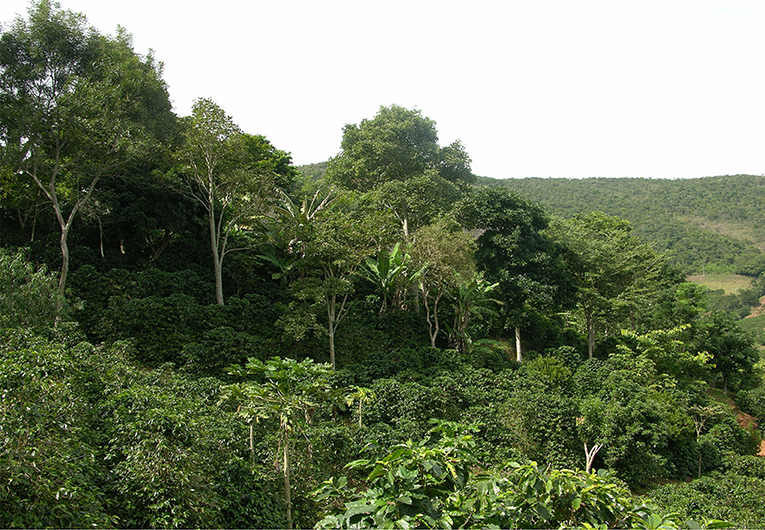The photograph captures a tropical jungle environment from a higher elevation, offering a sweeping view of lush, vibrant vegetation that extends endlessly to the horizon. The landscape is a sea of green, featuring an array of tall trees with slender trunks and branches, interspersed with bush-like trees that have waxy leaves. Some sections show a variation in the shades of green, with brighter and lighter hues reflecting the sunlight. To the left, there's a noticeable clearing where the vegetation is sparser, indicating either a cleared area or a pond. In the bottom right, there are brown patches that could be dirt or wood chips. A distant line of hills adds to the depth of the scenery. The sky above is clear and white, devoid of clouds, allowing the sunlight to shine through and illuminate the dense foliage below.